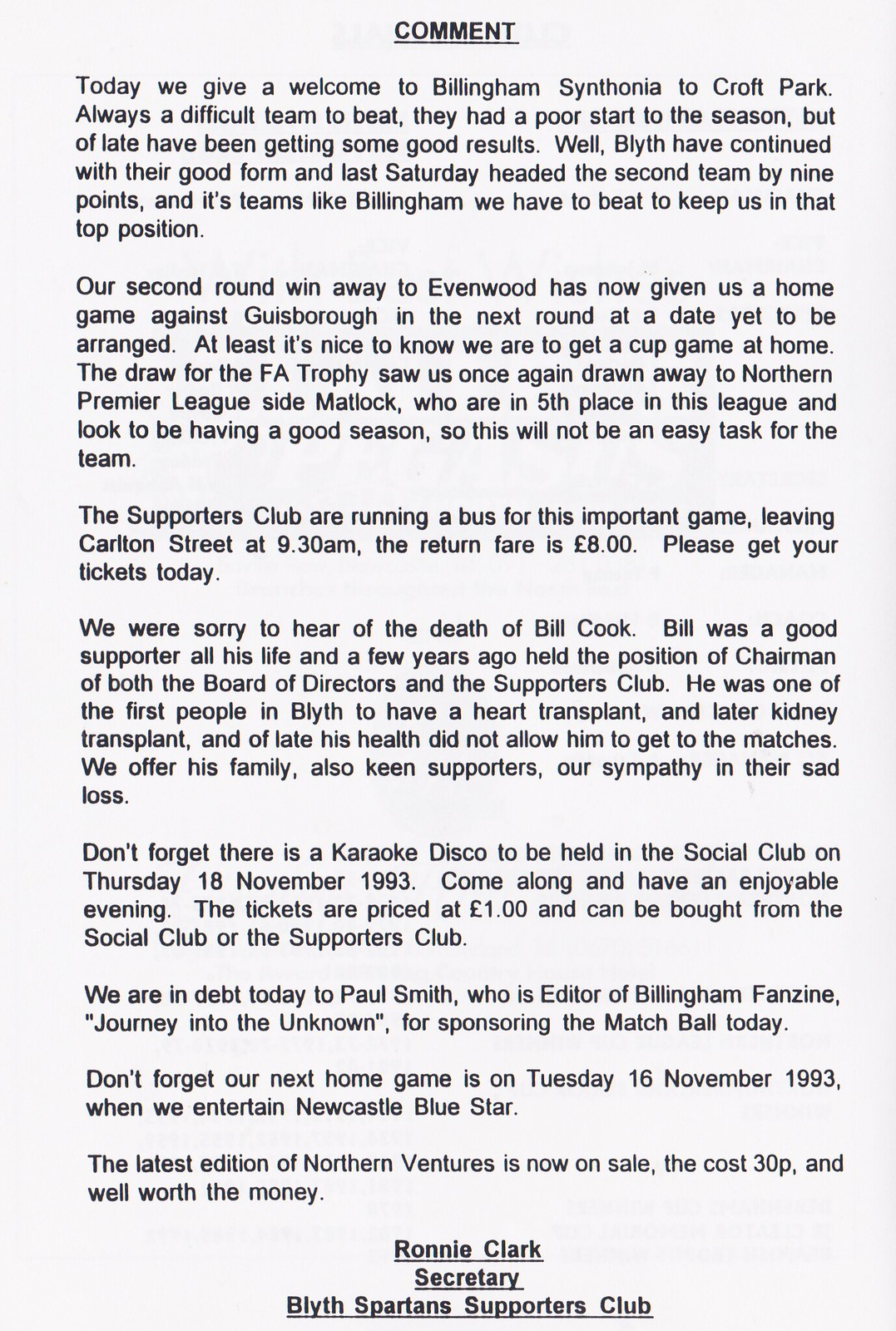The image is a notice on a white piece of paper with several paragraphs of text in black. At the top, underlined, it begins with "Comment." The text reads: 

"Today we give a welcome to Billingham Synthonia to Croft Park. Always a difficult team to beat, they had a poor start to the season, but lately have been getting good results. Meanwhile, Blythe have continued their good form and, as of last Saturday, lead the second team by nine points. It's teams like Billingham that we need to beat to maintain our top position.

Our second-round win away to Evenwood has now given us a home game against Guysboro in the next round, at a date yet to be arranged. The FA Trophy draw has us playing away against Northern Premier League side Matlock, who are in fifth place and having a good season. This will be a challenging match for the team. The Supporters Club is running a bus for this important game, departing Carlton Street at 9:30 AM with a return fare of eight pounds. Please get your tickets today.

We regret to inform you of the death of Bill Cook. Bill was a lifelong supporter and previously served as chairman of both the Board of Directors and the Supporters Club. Notably, he was one of the first people in Blythe to undergo a heart transplant and later a kidney transplant, though his health recently prevented him from attending matches. We extend our deepest sympathies to his family, who are also devoted supporters.

Don't forget there is a karaoke disco at the Social Club on Thursday, 18th November 1993. Tickets are priced at one pound and are available at both the Social Club and the Supporters Club. 

We are grateful to Paul Smith, editor of Billingham Fanzine 'Journey into the Unknown,' for sponsoring the match ball today. Don't miss our next home game on Tuesday, 16th November 1993, when we entertain Newcastle Blue Star. 

The latest edition of 'Northern Venues' is now on sale for 30p and is well worth the money. 

At the bottom of the notice, in bold print, it says: Ronnie Clark, Secretary, Blythe Spartans Supporters Club."